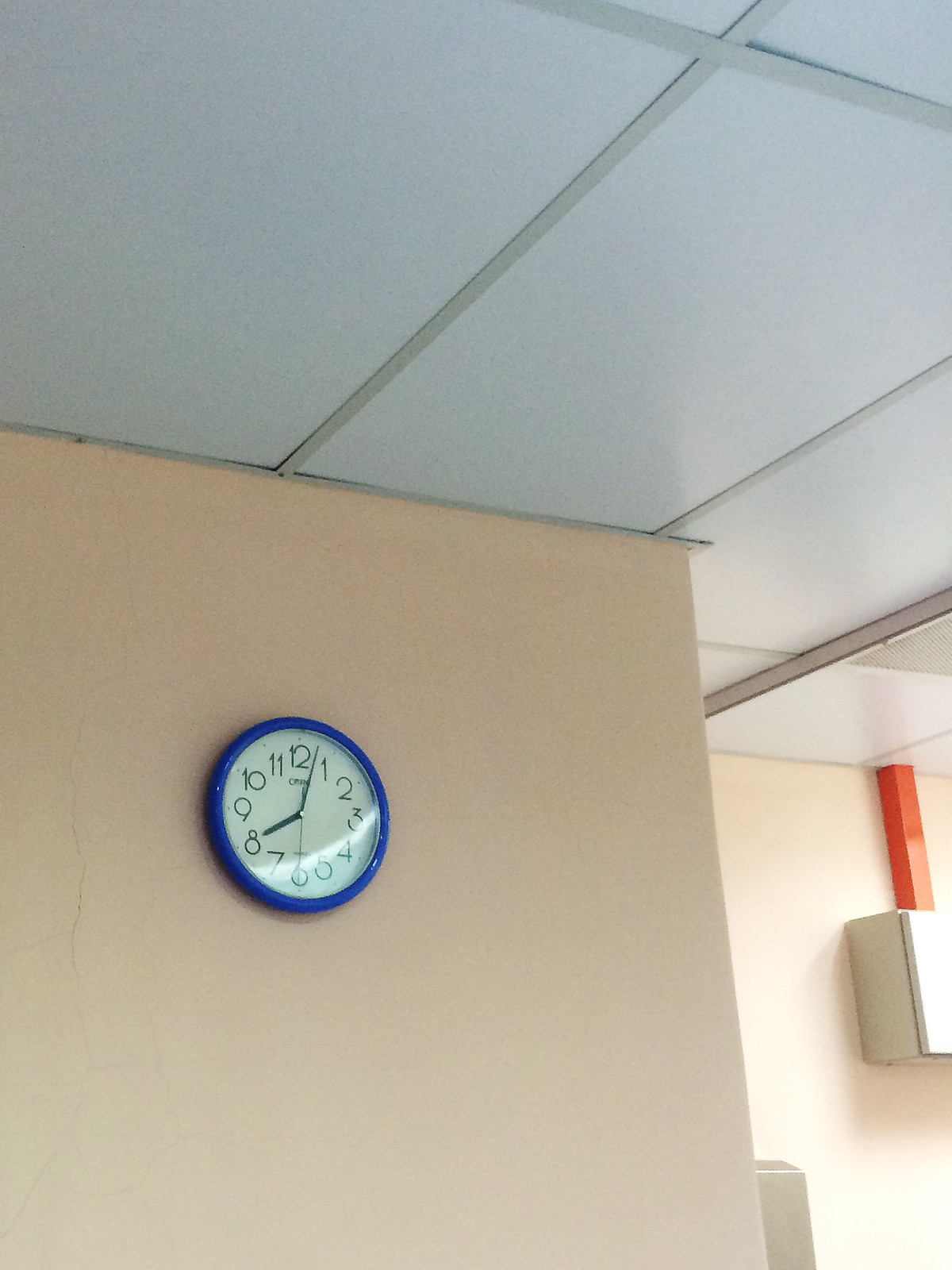In this photograph, we see a corner section of a wall, likely situated in an office or school building. The ceiling is composed of white and gray rectangular panels, each divided by thin lines. Toward the right of the image, a recessed wall features an orange and gray box, possibly housing an electrical or breaker unit. The main wall, painted a neutral tan color, is adorned with a small clock at its center. The clock is distinguished by a blue plastic outline and features a white face with numbers rendered in a decorative, curly font, capturing both functionality and style.